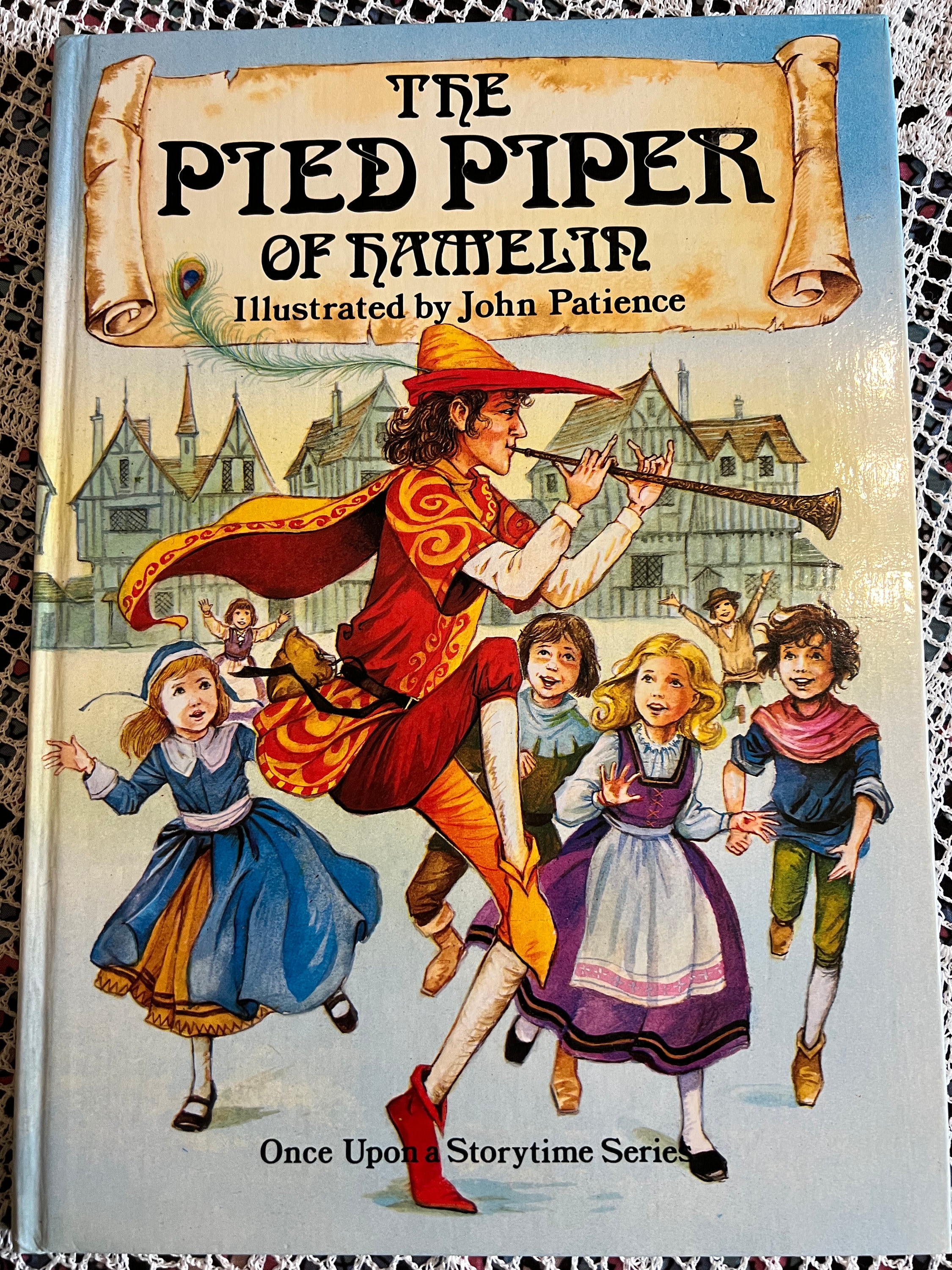This is a photograph of the cover of a children's book titled "The Pied Piper of Hamelin," illustrated by John Patience. The book is set on a black table covered with a white knit tablecloth, which is partially see-through. At the top of the cover, the title is written in black text on a yellow scroll. Below the title, there is an illustration depicting the Pied Piper playing a flute. He wears a yellow hat with a red brim and a long green feather, a red outfit adorned with gold designs, red and yellow shoes, and a red and gold cape. The Pied Piper stands with one leg lifted while playing his instrument. Surrounding him are numerous children, smiling and looking happy; some are wearing blue and purple dresses. In the background, there are illustrations of old Dutch-style buildings and large structures. At the bottom of the cover, the text reads, "Once Upon a Storytime Series."